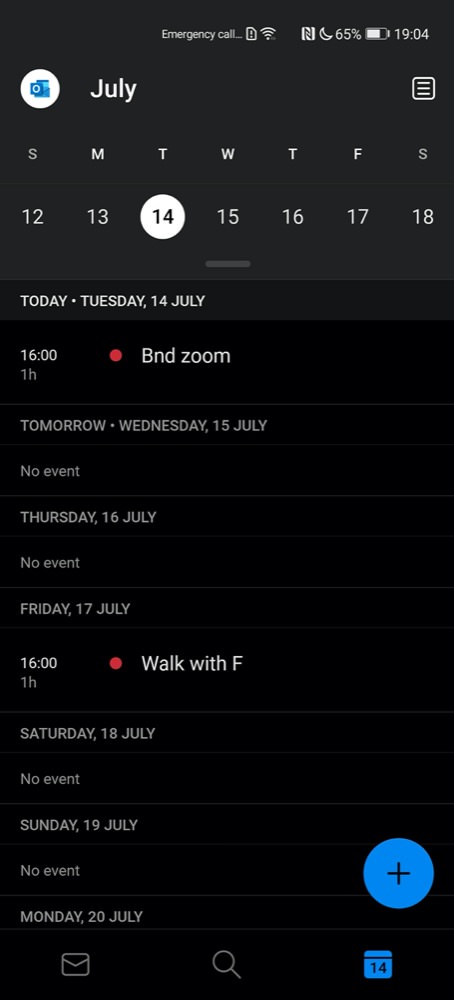The image shows a detailed view of a calendar and productivity app, likely Microsoft Outlook. At the top of the screen, there is an "Emergency Call" label with an exclamation point inside a rectangle. The status bar displays Wi-Fi signal strength, a moon icon indicating night mode, a battery level of 65%, and the time, 19:04.

In the main interface, the title "July" is prominently displayed alongside a white circle featuring the Outlook logo. A hamburger menu is located on the right. Below this header, the days of the week are abbreviated as S-M-T-W-T-F-S, spanning Sunday to Saturday. Beneath these abbreviations, the days of the month from the 12th to the 18th are shown in a sequential row. The current date, Tuesday the 14th, is highlighted with a white circle.

The section below this calendar grid details specific events for the week:
- On Tuesday, July 14th, an event is scheduled from 16:00 to 17:00 labeled "BND Zoom".
- On Wednesday, July 15th, there are no events listed.
- On Thursday, July 16th, there are no events listed.
- On Friday, July 17th, from 16:00 to 17:00, there is a "Walk with F," indicated by a red dot.
- On Saturday, July 18th, no events are listed.
- Sunday, July 19th, has no events shown.

The bottom of the screen includes navigation icons: a blue circle with a plus sign for adding new events and three other menu buttons for additional functionalities such as email (envelope icon), search (magnifying glass icon), and calendar view (calendar icon). The start of the next week, Monday, is not visible as it is off the bottom of the screen.